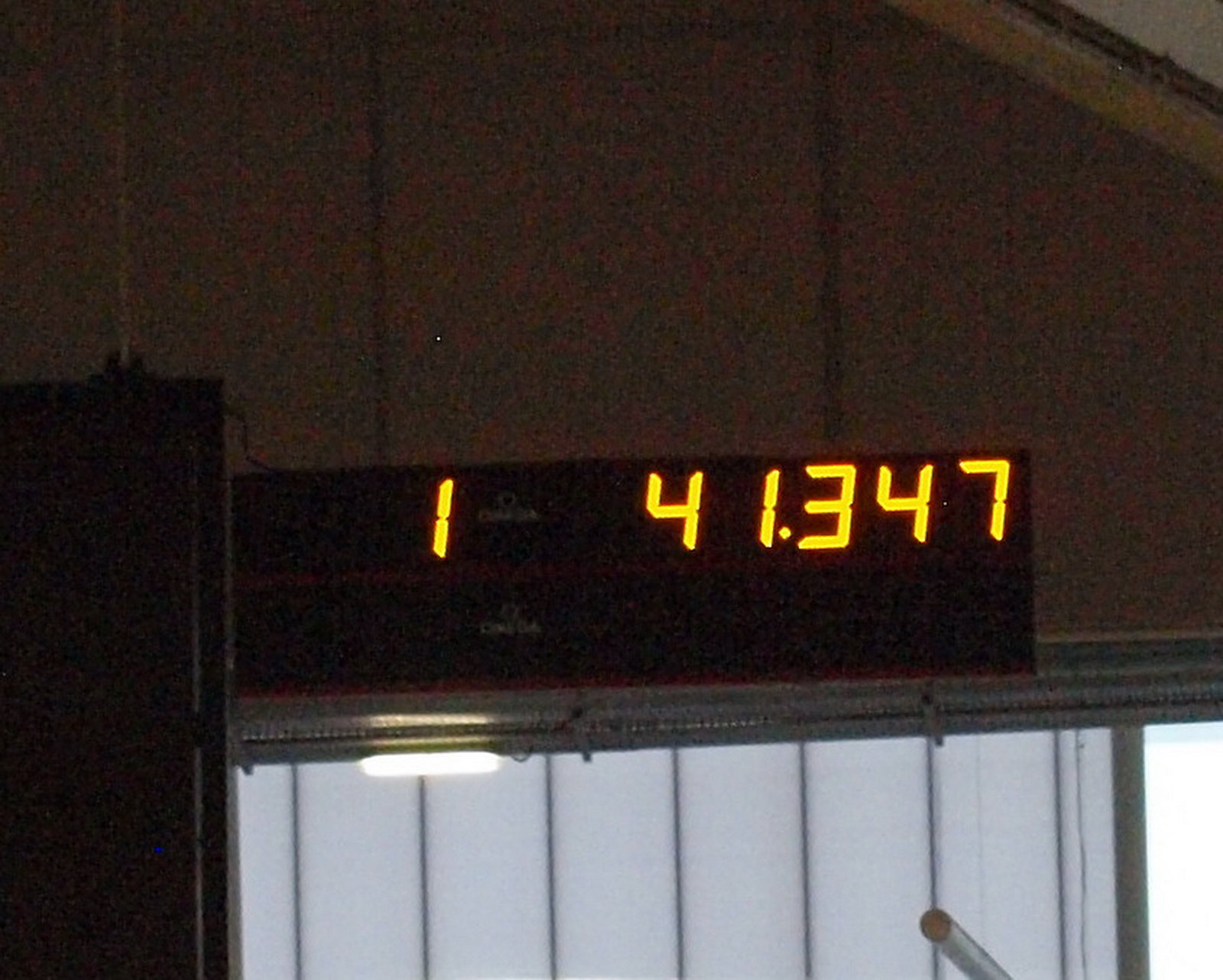A poorly illuminated color photograph features an enigmatic LCD display device adorned with barely discernible elements. The display is situated against a murky greyish or brownish wall. The foreground reveals a lighter grey section equipped with some metal bars, along with a small round diagonal bar positioned at the lower right-hand corner. To the left, there is a dark, shadowy area. The display itself has an indistinct yellow or red edge that is poorly rendered. The digits visible on the screen include a "1" on the far left, followed by "41.347," indicating that the display is not a typical clock but possibly some other kind of measurement device. Additionally, there is a small white dot located above the "1," situated in the middle of the brown wall area, which may or may not be a metallic object reflecting light.